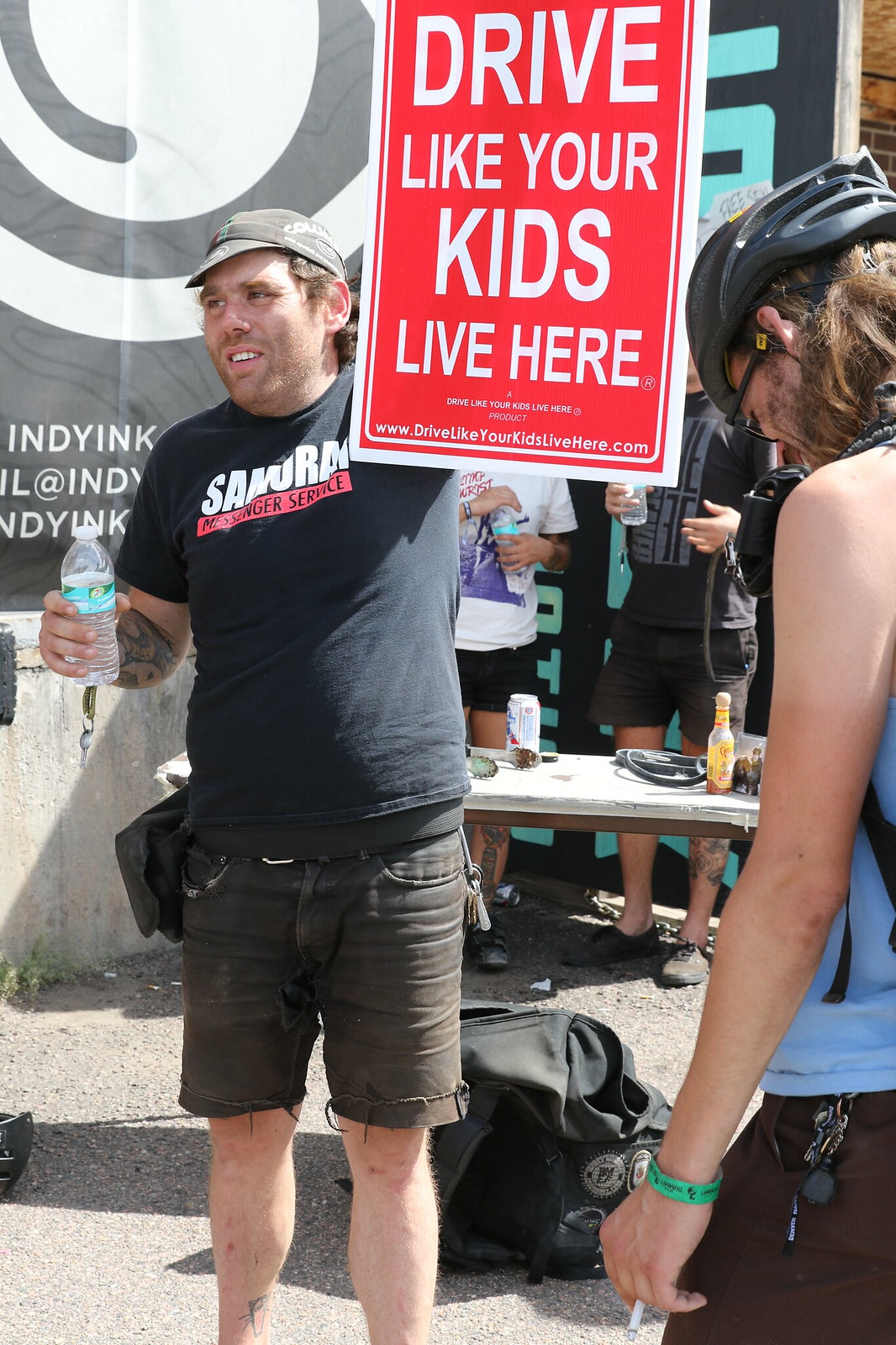The photograph captures a scruffy-looking man, reminiscent of a punk rocker, standing outdoors. He's dressed in a black t-shirt with "Samurai Messenger Service" emblazoned on the front and cut-off, dark olive shorts that fall just above the knee. He wears a black cap, has his hair tucked behind his ears, and sports a belt with a fanny pack. Tattoos adorn his right forearm and one shin. He holds a plastic water bottle in his right hand and a large red poster in his left, which reads "Drive Like Your Kids Live Here" in white text, along with the URL www.drivelikeyourkidslivehere.com. Standing to his right is a woman dressed in a light blue tank top, black pants, a green wristband on her wrist, and a black bicycle helmet on her head, looking downward. The background includes a table with assorted beverages and possibly hot sauce, other people dressed in bike gear, and a banner, all set on gravel, indicating a possible biking event or protest.